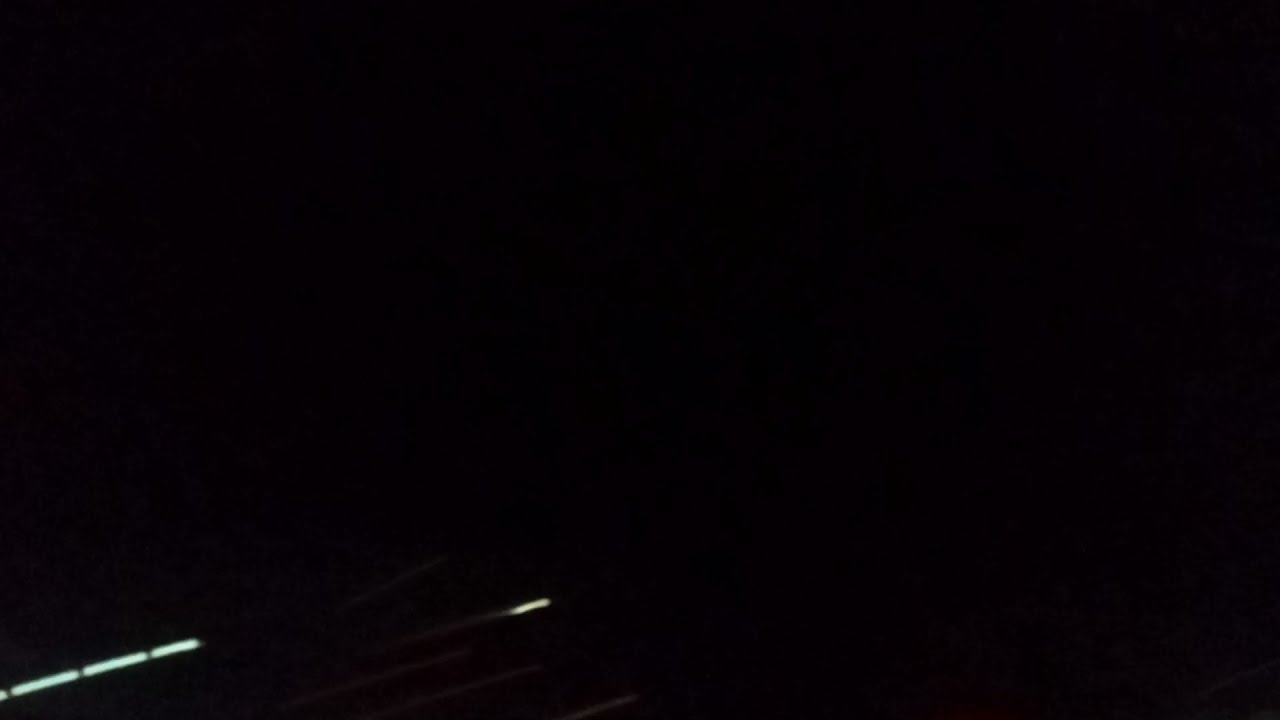The image is predominantly black, resembling either a piece of digital art or an extremely underexposed photograph, with its only discernible features located in the bottom portion. The bottom right corner of the image contains small, faint, elongated, rectangular shapes that might be interpreted as lights, one of which is a hint of a smudge of yellow, and a possibility of dull green. These lights or features are barely visible against the predominantly flat black backdrop. The bottom left corner displays thin strips of light, possibly white or grey, and resembles floor lighting that one might find in a dark movie theater. These thin strips are subtle, suggesting very dim illumination in an otherwise pitch-black image, while the entire setting appears devoid of any text or other colors beyond the grayscale tones and faint touches of yellowish light. This minimalistic composition can be seen as an abstract art piece or an accidental photograph taken in a very dark environment.